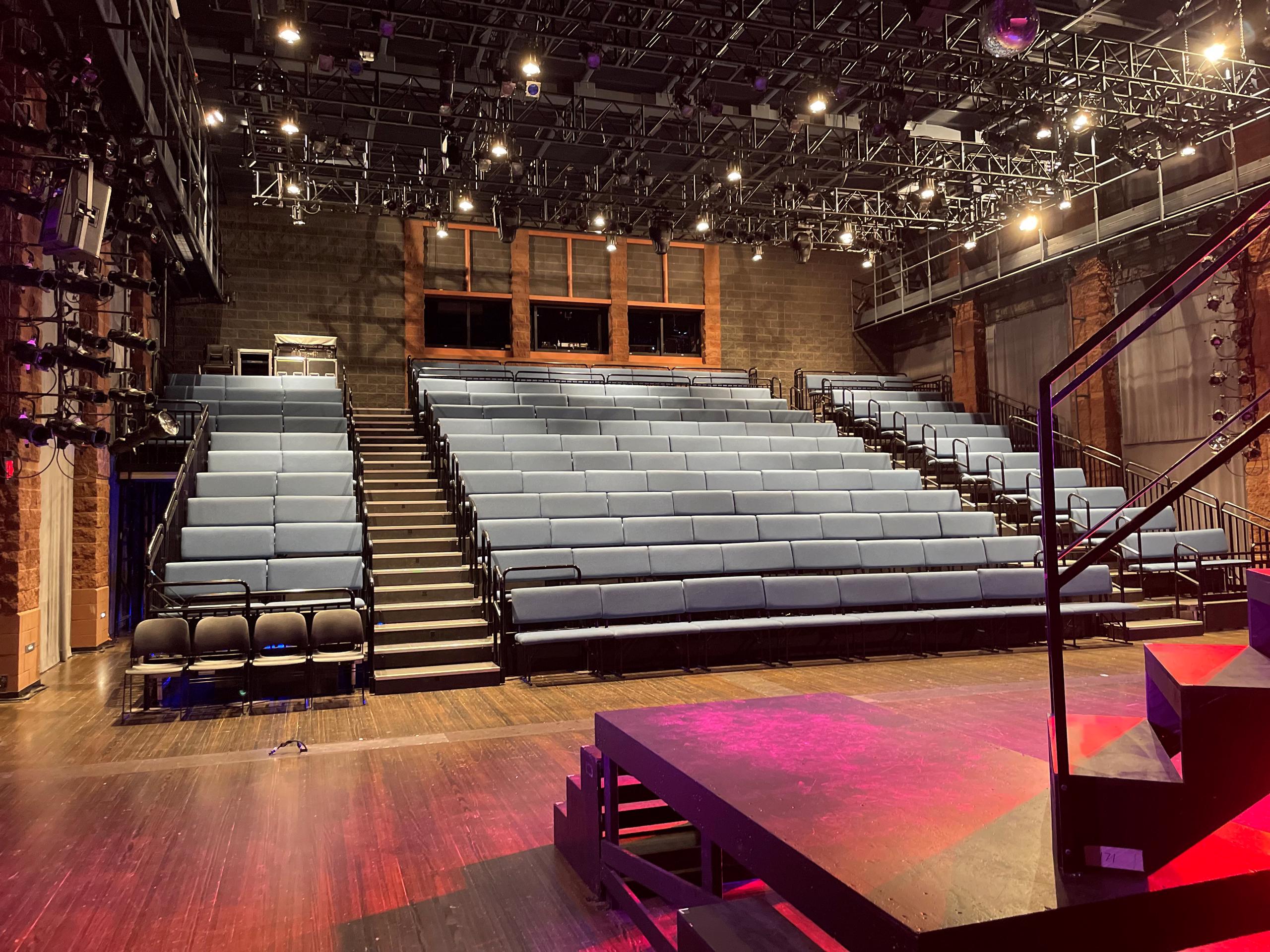The photograph captures a well-lit auditorium with a landscape orientation, featuring a stage and an array of seating. In the lower left-hand corner is a stage with a wooden floor and a raised black platform, equipped with stairs and hand railings on either side. The seating arrangement includes blue chairs divided into three columns: the left and right columns each containing approximately 2 seats per row, and the middle column housing about 10 seats per row, spanning around 15 to 20 rows. Staircases flanked by hand railings are positioned between the columns. The ceiling is fitted with metal scaffolding and extensive lighting fixtures, casting a bright ambiance over the space. The backdrop displays a brown brick wall adorned with three tall windows, while the side walls, also brick with windows, feature additional lighting. In the distance, there is a wooden camera box, and the auditorium is empty of people, emphasizing its intricate architectural details.